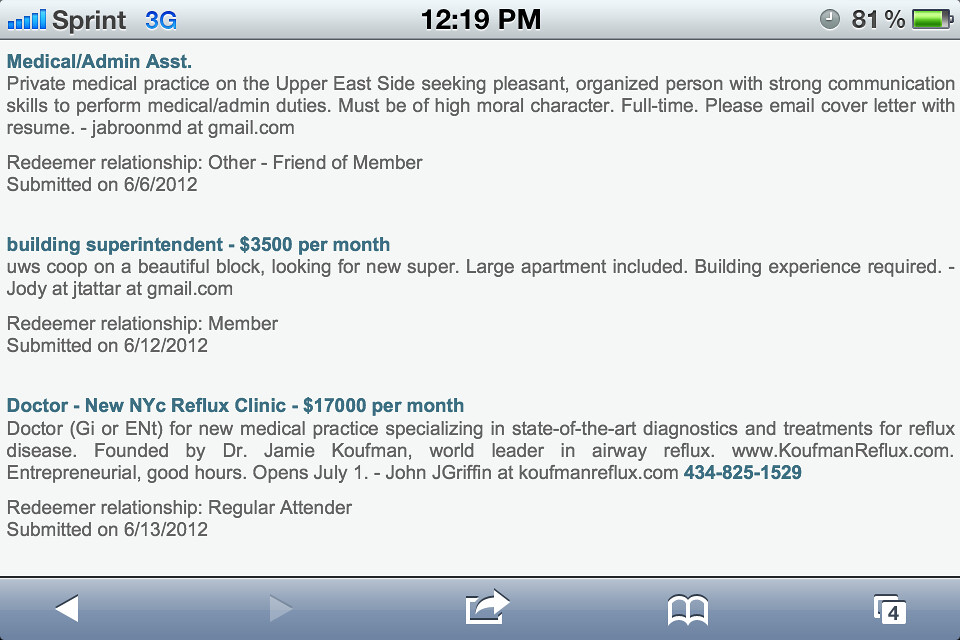This image is a screenshot of a web page displayed on a mobile browser. At the top, the notification bar shows a Signal icon on the left with "Sprint 3G" written next to it. In the center, the time is displayed as 12:19 PM, and on the right, the battery indicator shows 81% with a green battery icon. Below the notification bar, the web page contains job postings against a white background. The text for each posting is primarily in black, with headings in blue. The first job listing is for a "Medical/Admin Assistant" at a private medical practice on the Upper East Side, requiring strong communication skills and high moral character; applicants are instructed to email their cover letter and resume to jbroonmd@gmail.com. The second job listing is for a "Building Superintendent" offering $3,500 per month, which calls for building experience and a new super for a USW Coop; interested parties should email Jody at J-T-A-T-T-A-R at gmail.com. The third listing is for a "Doctor - New NYC Reflux Clinic" with a salary of $17,000 per month, detailing a new medical practice funded by Dr. Jamie Kaufman; contact details include a website, www.kaufmanreflux.com, and an email, john.j.g.griffin@kaufmanreflux.com, as well as a phone number, 434-825-1529. At the bottom of the screenshot, a horizontal bar contains icons, including back, forward, share, a book, and tabs icons.